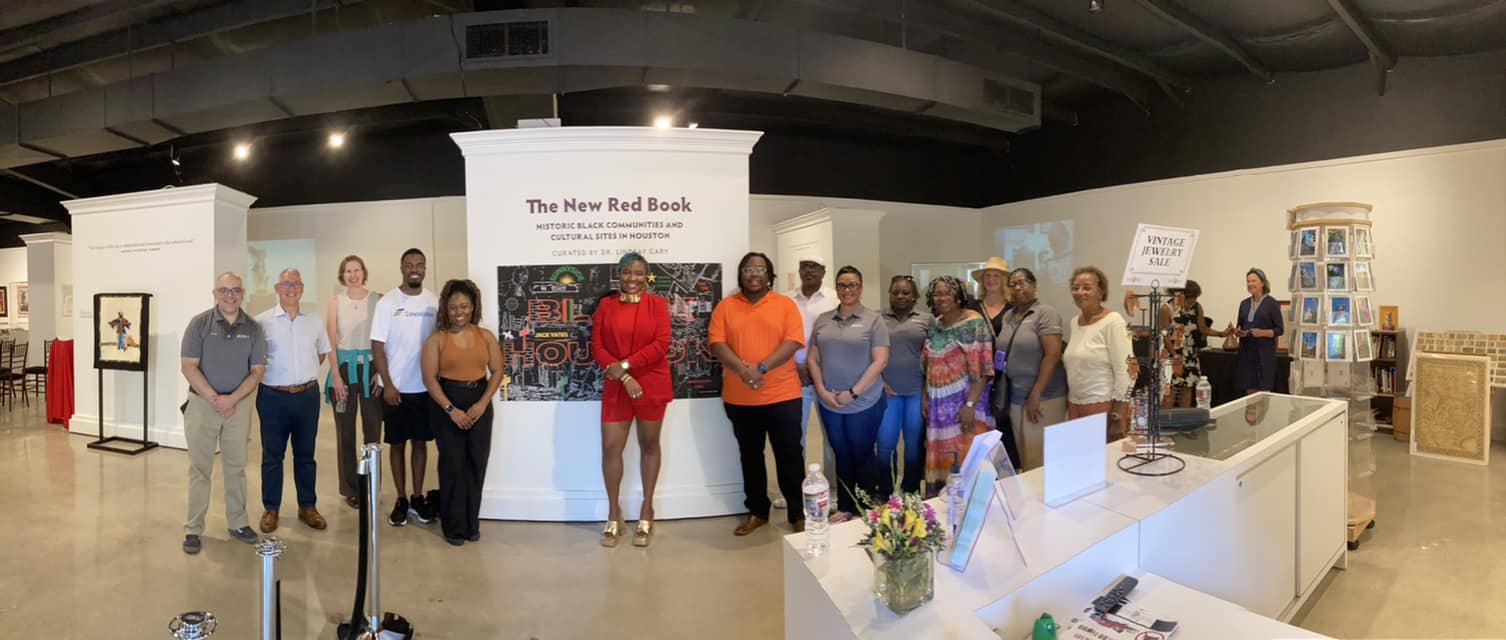This detailed panoramic color photograph captures a large group of around 15 to 20 people, predominantly Black with a few White individuals on the left side, smiling and posing together in what seems to be an art gallery or exhibition space. The center of the image features a white display with the exhibit's title in red text: "The New Red Book: Historic Black Communities and Cultural Sites in Houston." Below the main title, another poster with red and yellow text reads "Black Houston." The surrounding space has a modern feel, with a grey high ceiling and visible air ducts. In the foreground, on the right side, there's a white counter with a glass top, possibly for checking people into the museum or gallery. This counter also bears a white sign that reads "Vintage Jewelry Sale.” Additionally, a postcard stand is visible near this counter. The group poses on a brown floor, emphasizing the contemporary and clean atmosphere of the display area.